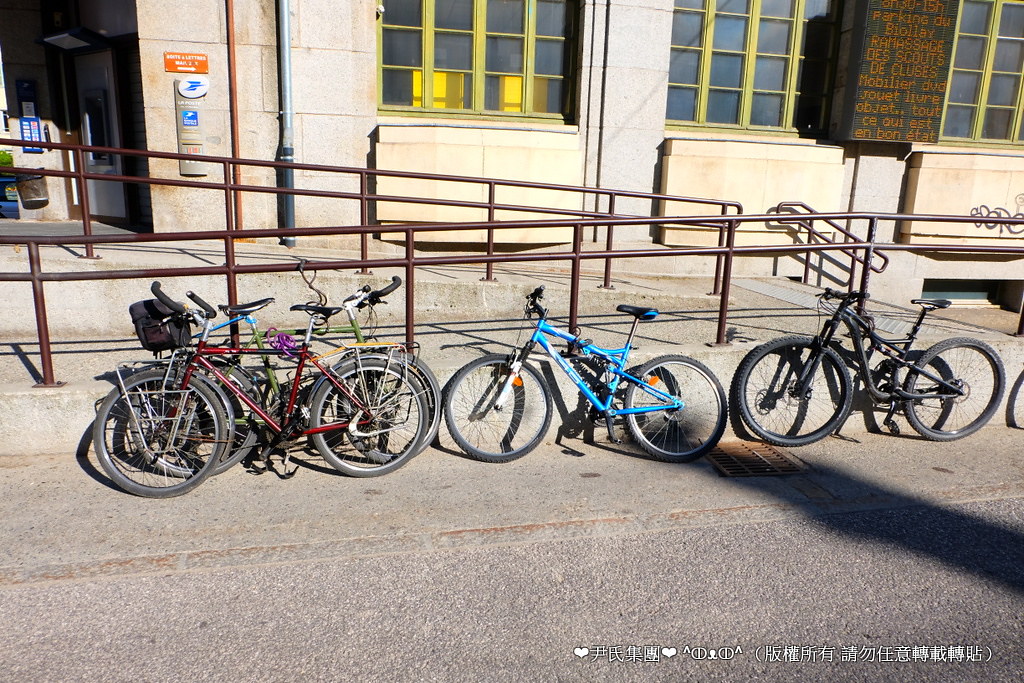The photograph captures a vibrant city street scene featuring a gray pavement sidewalk adjacent to the road, with multiple bicycles propped against a stone gray wall. There are at least four bicycles visible, including a green and a red bike leaning on each other, a light blue bike, and a black bike. These bikes appear to be mostly mountain bikes. The image also includes a series of metal railings and ramps, which seem smooth enough to accommodate wheelchairs. A metal stairway leads up one of the ramps. In the background, a tan brick building with windows partially painted yellow adds an architectural element to the scene. It's possibly a school building, as indicated by the window design and small glimpse of an entrance on the left. Symbols in another language are visible along the right edge of the photograph. The overall composition reflects an urban, accessible walkway with a mix of transportation and architectural details.